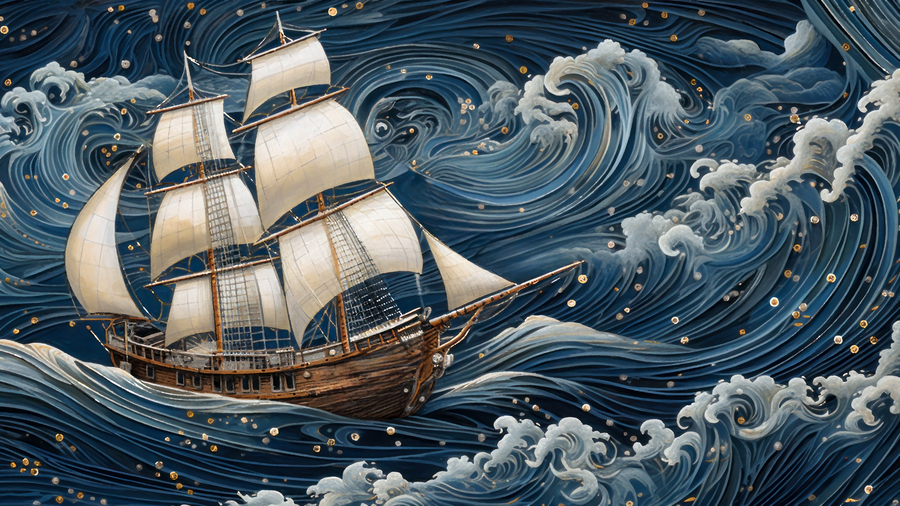This detailed illustration captures a large, wooden ship reminiscent of a vessel from the 1400s, similar to the Mayflower. The ship, with its brown wooden hull and cream-colored sails, is depicted sailing through a tumultuous, stylized sea. The ocean's waves are elegantly graphic, curving dramatically with shades of dark blue, light blue, and off-white. Gold-orange dots speckle the scene, adding a touch of fantasy. Despite the violent and exaggerated nature of the waves, the ship remains stable and unthreatened. This beautifully painted image, evocative of a children's book illustration, combines elements of historical and fantasy styles to create a timeless seafaring adventure.